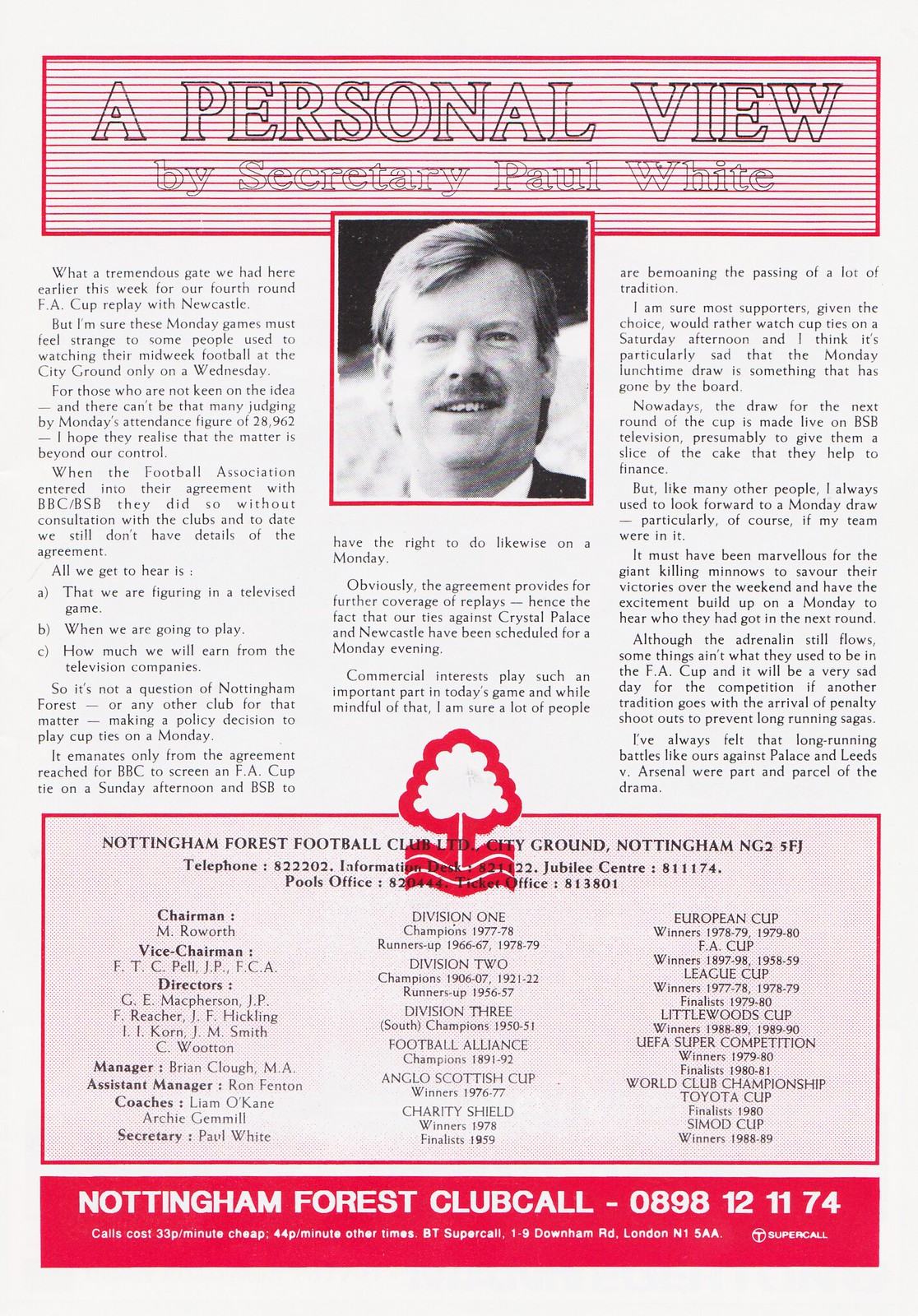The image is a page from a magazine or booklet. At the top, within a pink box outlined in black, the large letters "A" and "PERSONAL" are prominently displayed. Below, in faint text, it reads: "A personal view by Vice Secretary Paul White." Accompanying this text is a black and white photo of Paul White. Further down the page, a logo featuring a tree, outlined in red, is present. Beneath this logo, the text "Nottingham Forest Club Hall-0898-12-1174" is visible. Additional small print at the bottom reads: "Coles Cross. 3-5-P-Minute-Cheap. 44-P-Minute-Other-Times. 8-T-Super-Call. 1-9-Downham Road, London. N15AAA." The article includes detailed small prints and logos, and in a box in the middle, it states: "Nottingham Football Club. Limited city ground, Nottingham," providing membership information. This personal narrative by Secretary Paul White outlines the challenges and opinions regarding scheduling changes for FA Cup replays, noting the high attendance of 28,962 for a Monday game against Newcastle. White also discusses the lack of consultation from the Football Association regarding broadcast agreements with BBC and BSV, emphasizing the need for clubs to have more input in such decisions.